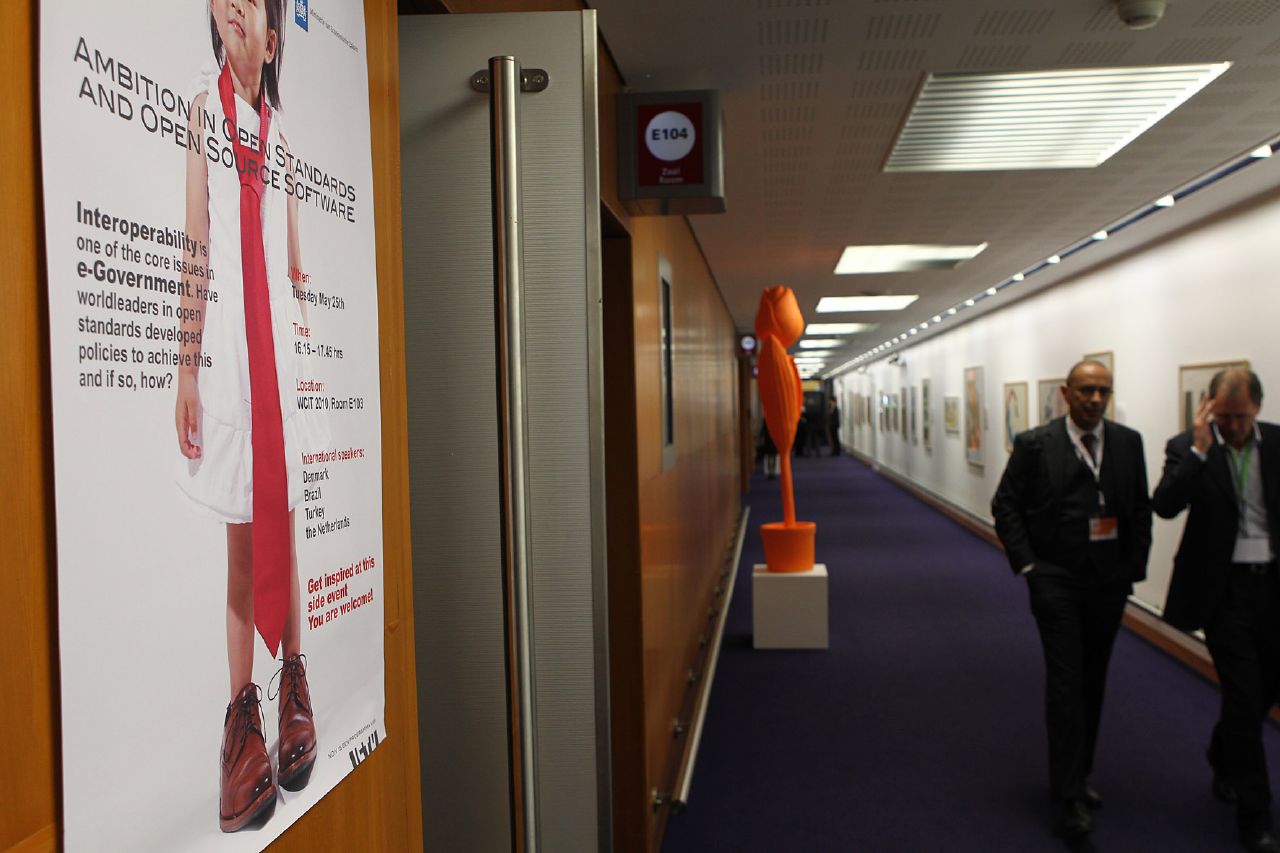The image depicts an indoor corridor in a building, extending into the distance with a blue carpet underfoot. The walls are a combination of white and wood; the right wall is white and adorned with a multitude of photographs, while the left wall is wooden. Fluorescent lights, including square panel lights and small dot lights, provide illumination from the ceiling above.

Directly to the left, a prominent poster features a young girl dressed in a red tie, white dress, and oversized men's brown shoes. The poster contains extensive text, including a notable headline: "Ambition in Open Standards and Open Source Software" and additional informational text about e-government interoperability and its core issues. Other segments of the poster mention the date "Tuesday, May 15th" and a timeframe, "6.15 to 5.45."

In the scene, two men walk towards the camera. The man on the left is balding with a black blazer, white shirt, and a green lanyard; he has his hand on his head, glancing downwards. The man on the right, bald with brown skin and glasses, has his hands in his pockets and is looking towards the camera. Both are wearing lanyards with badges.

To the left, beyond these men, an orange sculpture resembling a flower in a pot is displayed on a white pedestal. Above this area, a lighted box labeled "E-104" is mounted near the ceiling with unreadable text below it. Further in the distance, the corridor appears busy with many more people visible.